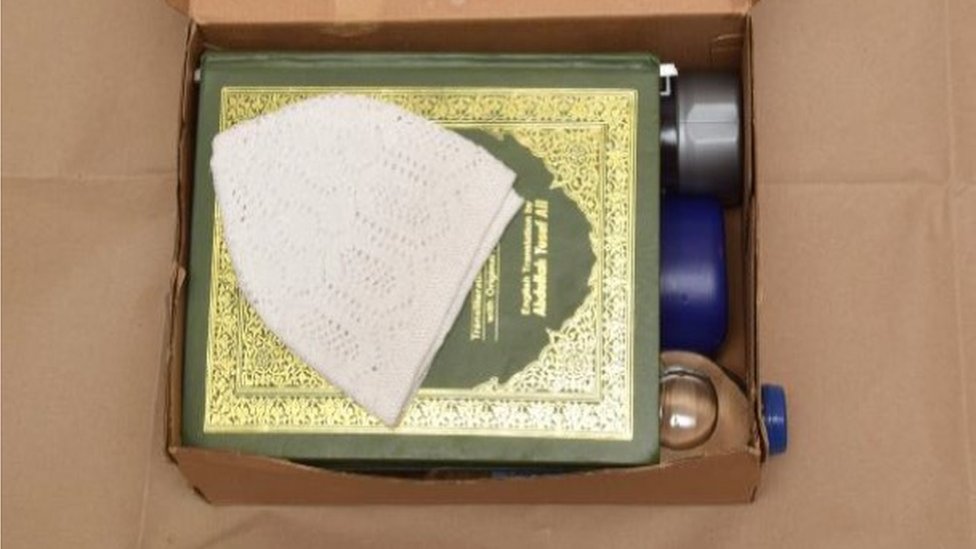The image features a horizontally rectangular open cardboard box, centrally positioned on a brown, potentially cardboard or light tan tablecloth background. Inside the box, prominently displayed, is a dark green hardbound book with intricate gold details and unreadable gold lettering. Resting atop the book is a white crocheted or lace hat, triangular in shape with wide sides. Partially visible beneath the book are the tops of at least two cylindrical objects, likely water bottles—one with a silver lid and the other with a blue screw-on cap. In the lower right-hand corner of the box, a small blue bottle cap is standing upright. The scene appears to be set on a table, presumably in a domestic setting. The color palette of the image includes shades of brown, green, gold, white, black, blue, and clear.